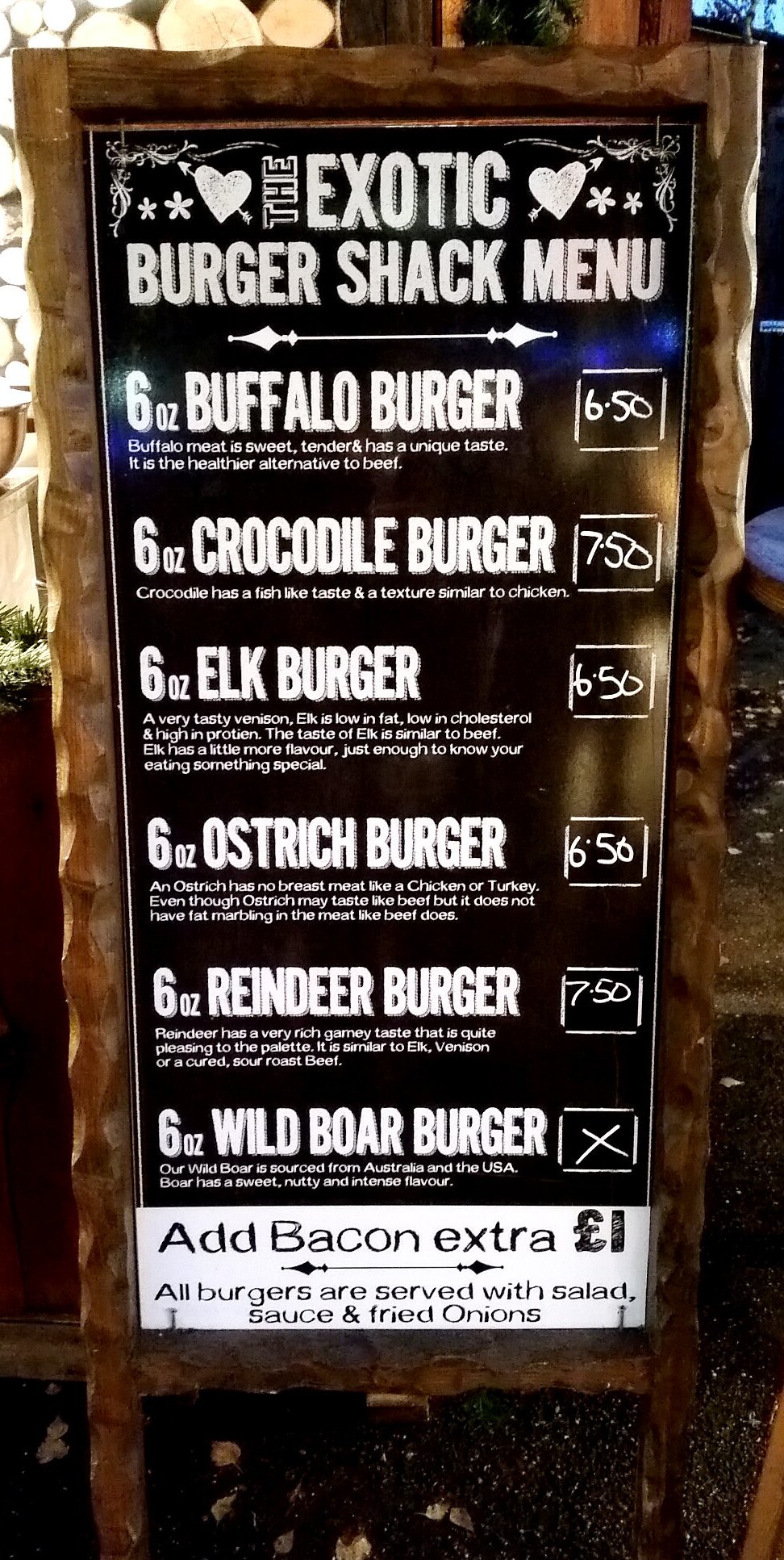The image features an upright rectangular menu board prominently displayed at the entrance of a restaurant, likely designed to catch the eye of incoming patrons. This menu board is set within a large wooden frame that is not perfectly straight; instead, it boasts a rustic and jagged appearance, featuring bumps and curves that give it a handcrafted, rugged charm. The wood extends all the way to the ground, lending a substantial and permanent feel to the structure.

Inside the wooden frame, the menu itself is presented on a black background. The setting around the menu appears to be somewhat dim, suggesting that it might be evening. Faint lights and patches of greenery can be seen in the background, and a hint of blue sky in the upper right corner indicates the waning daylight. Overall, the ambiance is intimate and slightly shadowy, emphasizing the illuminated menu text.

The menu is titled "The Exotic Burger Shack Menu" in bold white letters, with a decorative line and small arrows accentuating the title. Below the title, various exotic burger options are listed, each described in detail. The menu includes:

- A six-ounce buffalo burger
- A six-ounce crocodile burger
- A six-ounce elk burger
- A six-ounce ostrich burger
- A six-ounce reindeer burger
- A six-ounce wild boar burger

Each burger option includes a brief description of its ingredients and is accompanied by the price, which is enclosed in a rectangle for clarity. At the bottom of the menu, an additional note in white text with black lettering offers the option to add bacon for an extra dollar. It also states that all burgers are served with a side of salad, sauce, and fried onions.

This thoughtfully designed menu board serves as a striking and informative welcome to guests, enticing them with unique and exotic culinary options as they enter the restaurant.